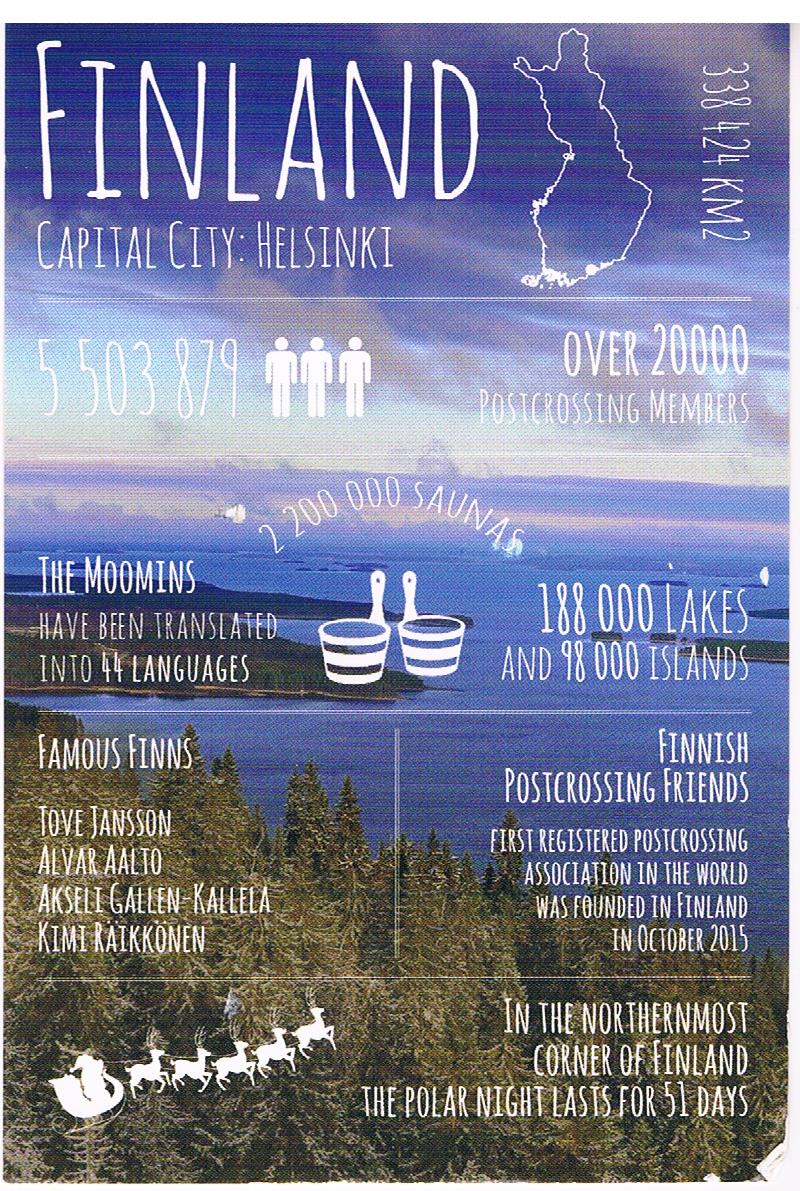This educational poster about Finland features a stunning background image of a scenic Finnish landscape, complete with calm waters, dense forests of pine trees, and a clear blue sky dotted with clouds. Overlaid in white text, the infographic includes key facts and statistics about the country. The title "Finland" is prominently displayed along with an outline of the nation’s map. Important geographical and demographic details are highlighted, such as the capital city, Helsinki, and Finland's size of 338,424 square kilometers. The population is listed as approximately 5.5 million people. Remarkably, Finland boasts 188,000 lakes, 98,000 islands, and 2.2 million saunas. The infographic also notes that the country has over 20,000 post-crossing members and features famous Finns like Tove Jansson, Alvar Aalto, and Kimi Räikkönen. Additionally, it mentions that a post-crossing association was founded there in October 2015. Adding a whimsical touch, a small white graphic of Santa Claus and his reindeer is included, accompanied by a note that in the northernmost corner of Finland, the polar night endures for 51 days.